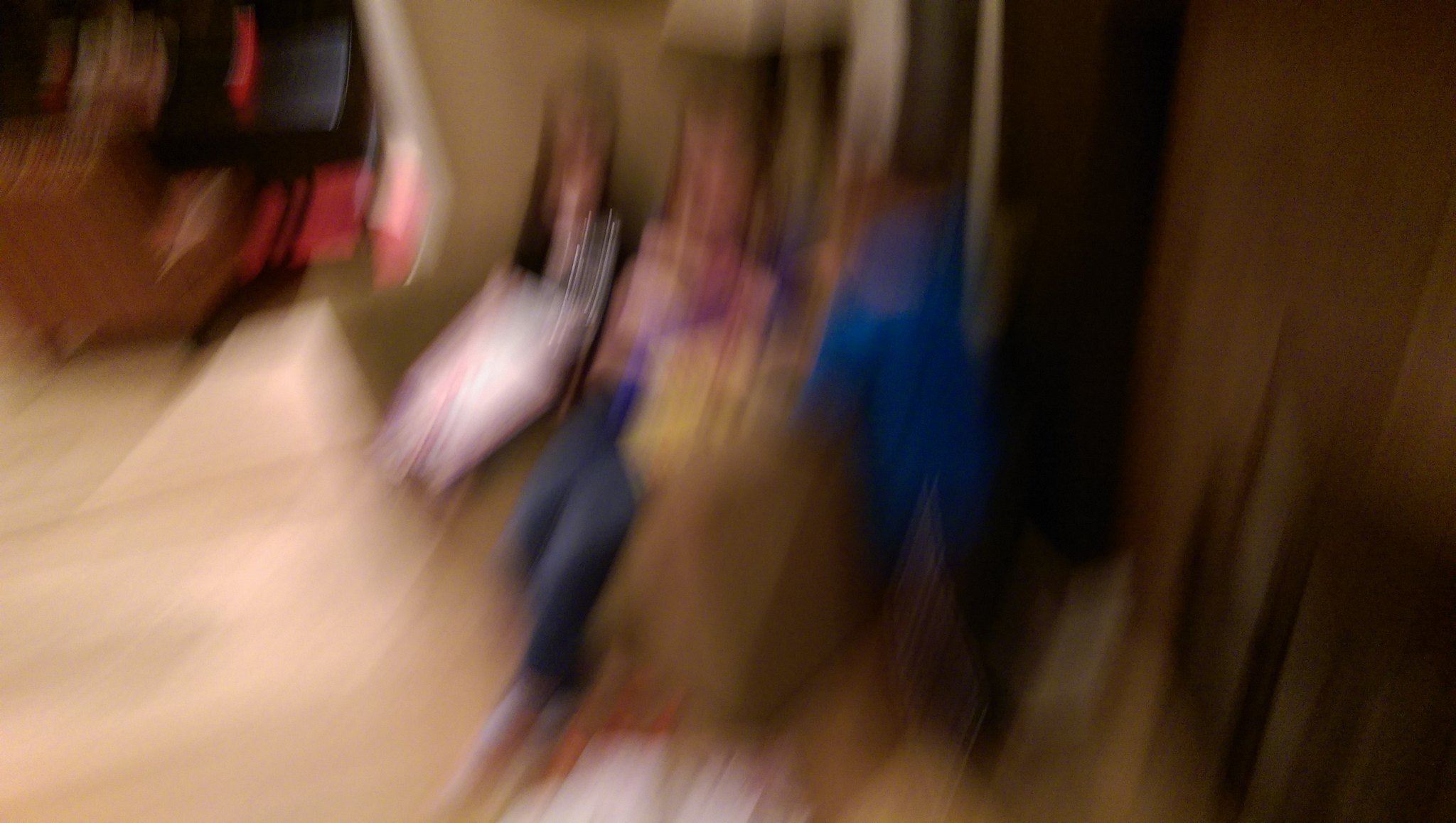This exceedingly blurry photograph, taken in a room with dark-colored walls, depicts three indistinct shapes that appear to be people, positioned centrally on a light-brown, possibly wooden floor. At the forefront stands a smaller child, clad in dark pants and a blue top. To the right, possibly seated, is a figure in a pinkish shirt with blue jeans. Adjacent to them is another person, characterized by a dark top and either pinkish bottoms or an item of the same color on their lap. The image also contains a doorway on the right side and displays an array of colors including blue, pink, black, and some reds and whites scattered on the ground.